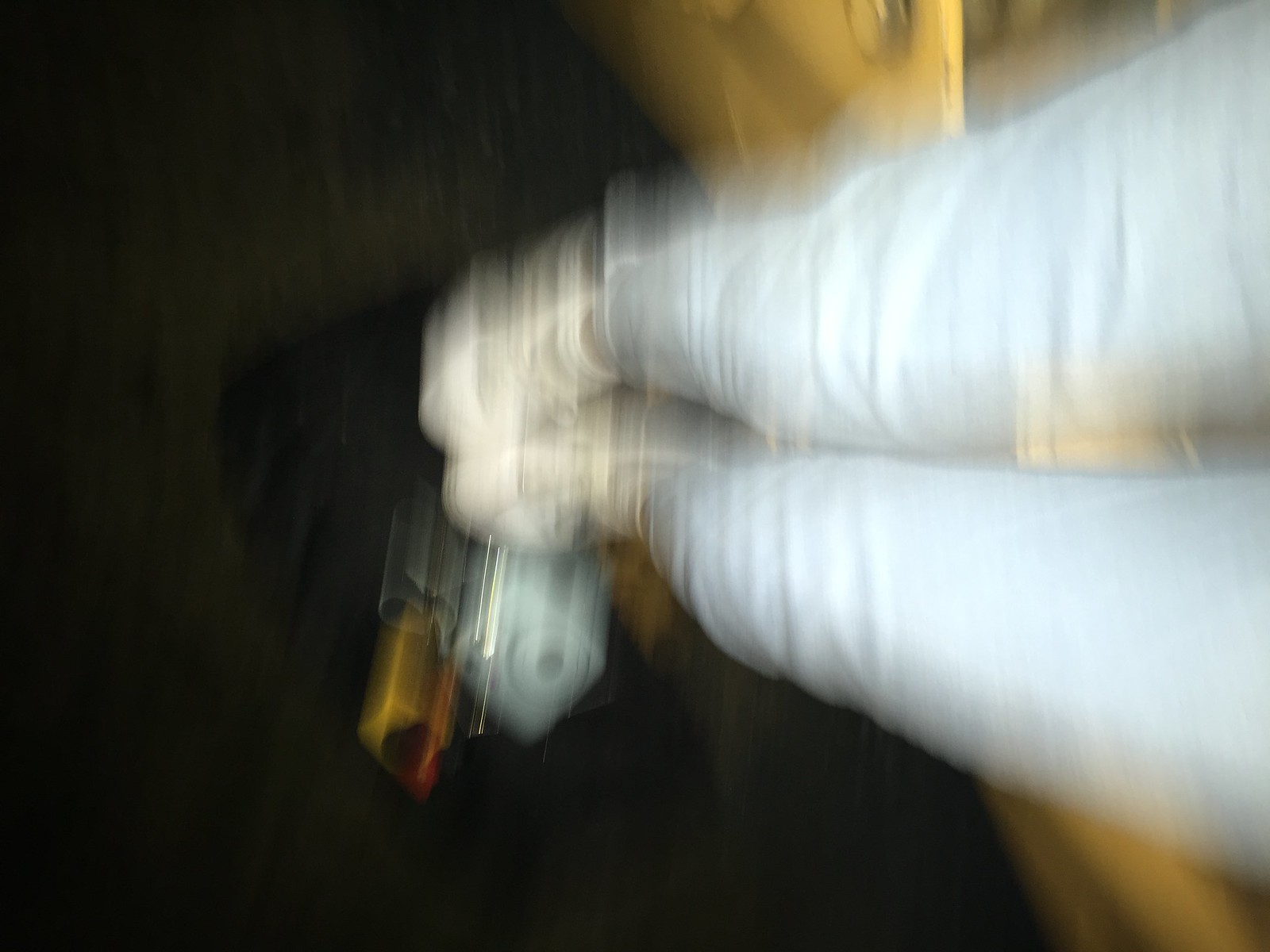The photo, despite its blurry quality, captures a pair of legs wearing tight, white pants and white sneakers standing on a dark floor, possibly black or gray concrete. The feet are pointing towards the left, with a white-gray Polaroid camera positioned to the left and slightly underneath the feet, lens facing up. This scene appears to be taken outdoors, likely at night, illuminated by a street light. Behind the legs, a yellow object is faintly visible, possibly indicating a difference in elevation or a structural element like a bench or car part. The image also contains additional objects near the feet: a red and orange item and a black tray or mat. Motion blur extends vertically through the image, making it challenging to discern finer details.